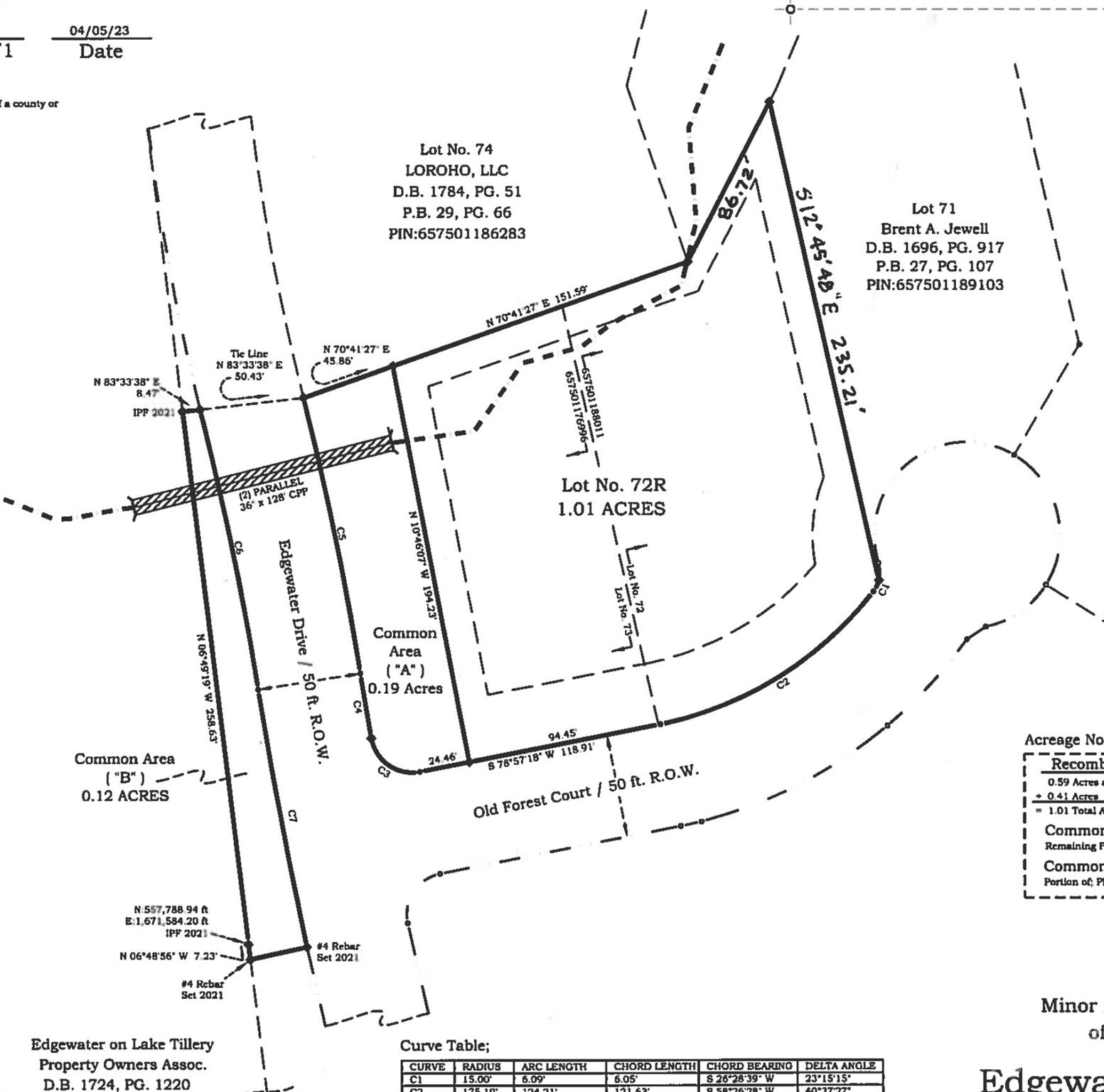This black-and-white property diagram depicts multiple lots within a specific area. In the upper left corner, the date "04-05-2023" is prominently noted. Central to the image is lot number 72, marked as 1.01 acres, flanked by various lots including lot 71 to the right, labeled "Brett A. Jewell, DB 1696, PG 917, PB 27, PG 107, PIN 657501189103." To the right of the central lot is a common area marked "Common Area" and "Old Forest Court 50-foot ROW," alongside "Edgewater Drive 50-foot ROW." The upper side of the diagram highlights lot number 74, labeled "Laura Ho LLC," while at the bottom, "Edgewater on Lake Tillery Property Owners Association, DB 1724, PG 1220" is inscribed. The diagram is detailed with varying line types—solid and dashed—demarcating property boundaries, building areas, and common spaces. A curved table with partially visible numbers is present at the bottom, indicating further data associated with the lots.